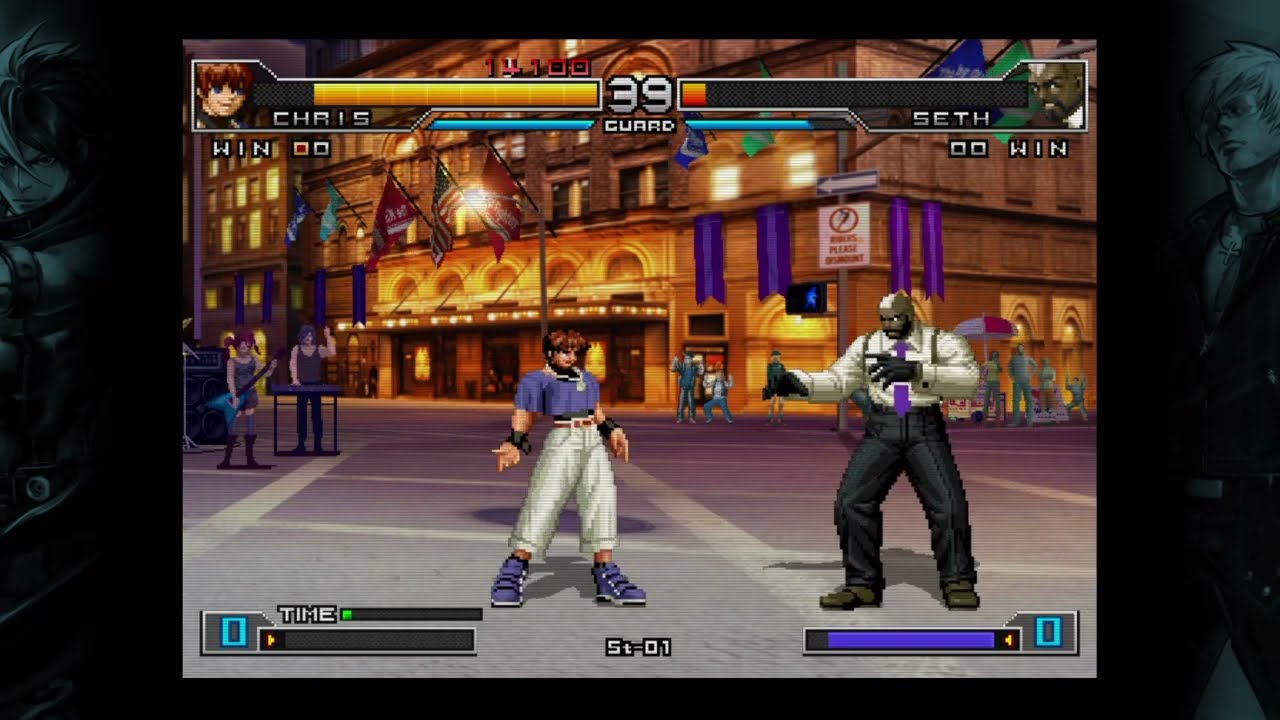The screenshot depicts an intense moment from a retro 2D fighting game, possibly from the battle royale or fighting genre akin to King of Fighters or Street Fighter. The scene showcases two distinct characters facing off. On the left is Chris, a younger fighter with short-cropped hair, wearing a blue shirt, white baggy pants, blue sneakers, and wristbands. He appears to be on the winning edge, with a life bar that is nearly full and a score of 14,1000. On the right stands Seth, an older, large black man with a blonde mohawk. Seth is dressed in a white shirt, black trousers, suspenders, black gloves, and a purple tie, evoking a professional or security guard persona. His life bar is significantly depleted, suggesting he is close to defeat. The backdrop features a large building and spectators gathered to watch the duel. The screen displays life bars, a power meter, scores, and round wins at the top, encapsulating the vibrant and competitive atmosphere.